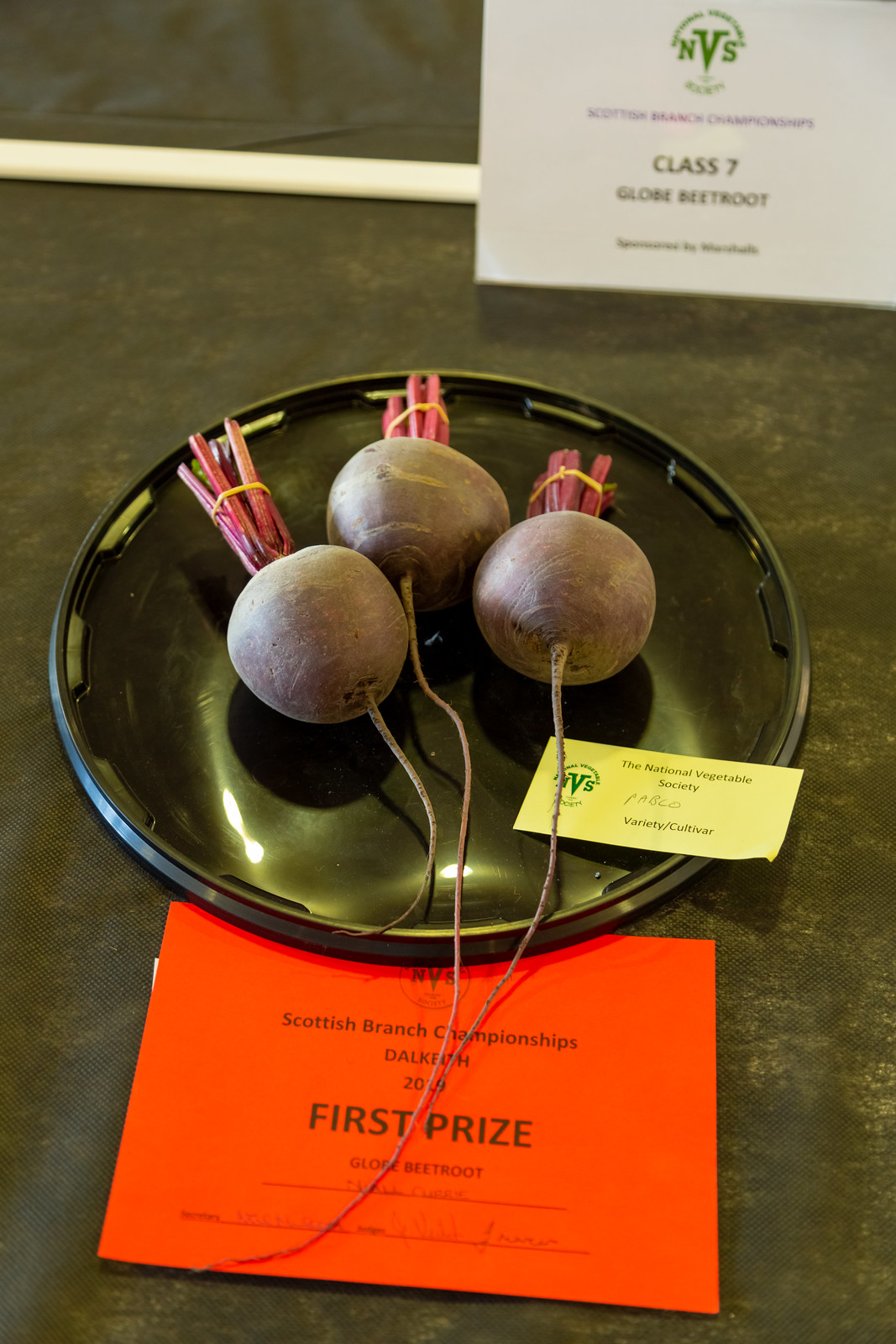This vibrant, full-color photograph showcases a green table with three purple beetroot globes garnished with stringy roots and topped with pink stems, all arranged in a bowl. To the top right of the bowl, a white placard prominently displays "NVS" in green, indicating the National Vegetable Society, and references the "Scottish Branch Championships, Class Seven, Globe Beetroot." Another small white card is seen partially obscured beneath the third beetroot. At the base of the bowl, an orange card with bold black print confirms the accolades: "Scottish Branch Championships, Dalkeith 2019, First Prize, Globe Beetroot." The image captures not just the beetroots but the recognition of their superior quality, suggesting they are of the 'Pablo' variety cultivar, celebrated for their perfection at the event.